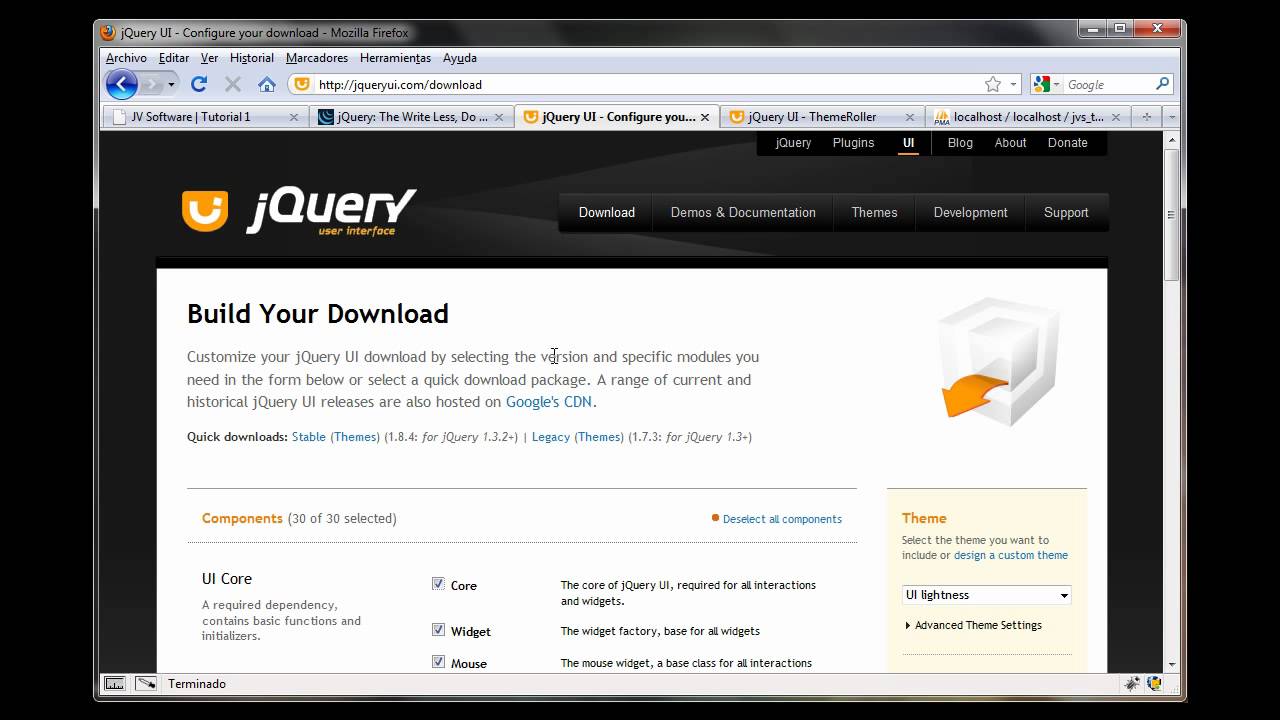This image is a screenshot captured from a Firefox web browser displaying the website https://jqueryui.com/. The browser's background is entirely black, and the top bar reads "jQuery UI: Configure Your Download – Mozilla Firefox." There are five tabs open, titled "JV Software Tutorial," "Query the Right Less," "jQuery UI: Configure Your Download," "jqueryut," and "localhost."

The website shown has a striking black background and features the "jQuery User Interface" header accompanied by a distinctive yellow and white logo with a curved "J." Below this header, there are several navigation buttons displayed, labeled "Download," "Demos and Documentation," "Themes," "Development," and "Support." 

The central content area of the website contrasts with a white background and provides instructions under the heading "Build Your Download," written in black text.